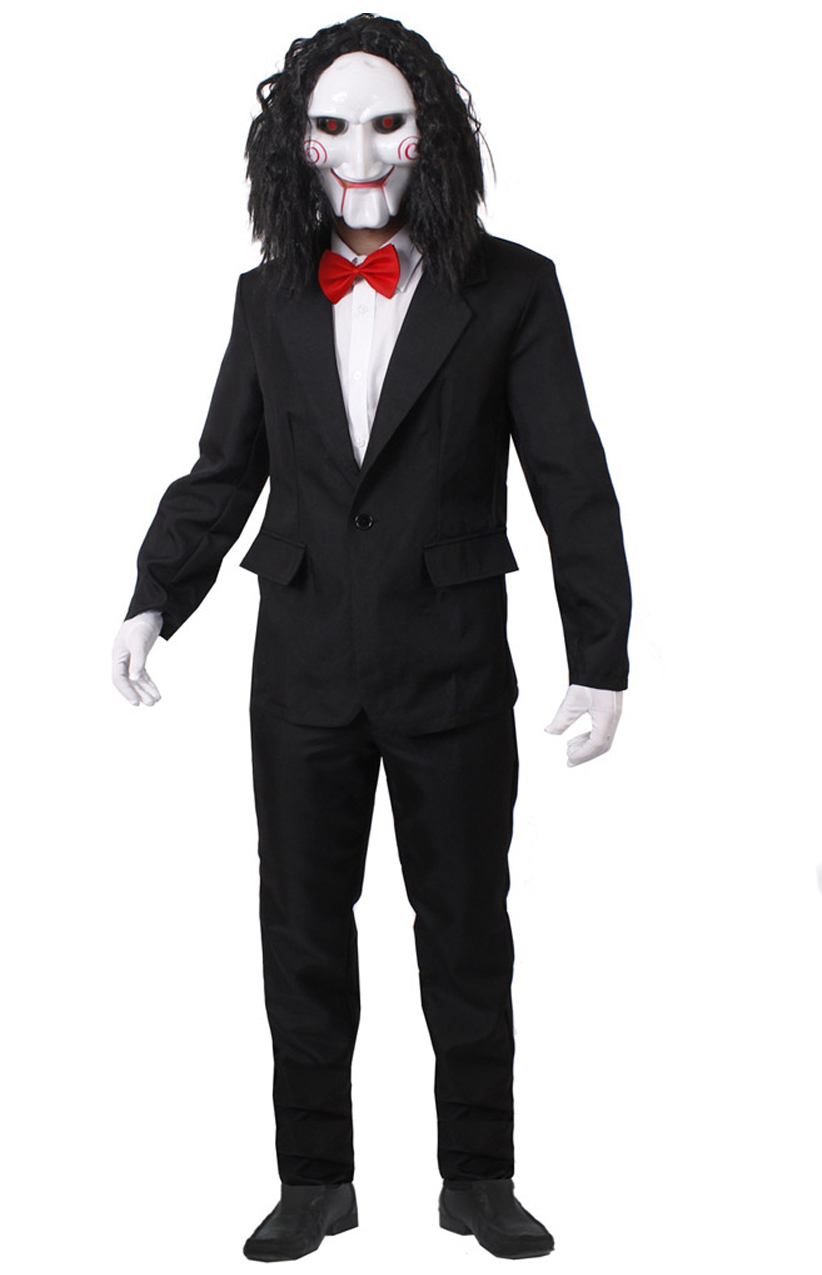This is a detailed product photo of an adult Halloween costume featuring a person dressed as Billy the Puppet from the Saw movies. The individual is standing upright against a completely white background, which accentuates the costume's details. They are donning a black tuxedo jacket paired with matching black pants and black shoes. Their attire includes a white button-down shirt underneath the jacket, accentuated with a red bow tie at the center of the collar. White gloves cover their hands, complementing the white shirt and adding to the overall eerie aesthetic.

The focal point of the costume is the iconic Billy the Puppet mask. The mask features a stark white face with red swirls on the cheeks, giving it a distinctive menacing look. It has black scleras with red irises, and a slender, red-lipped smile that is reminiscent of a skull. Completing the grotesque visage is wiry, shoulder-length black hair that drapes around the sides of the mask, enhancing the sinister appearance. This costume perfectly captures the chilling essence of Billy the Puppet, making it a standout choice for any horror-themed occasion.